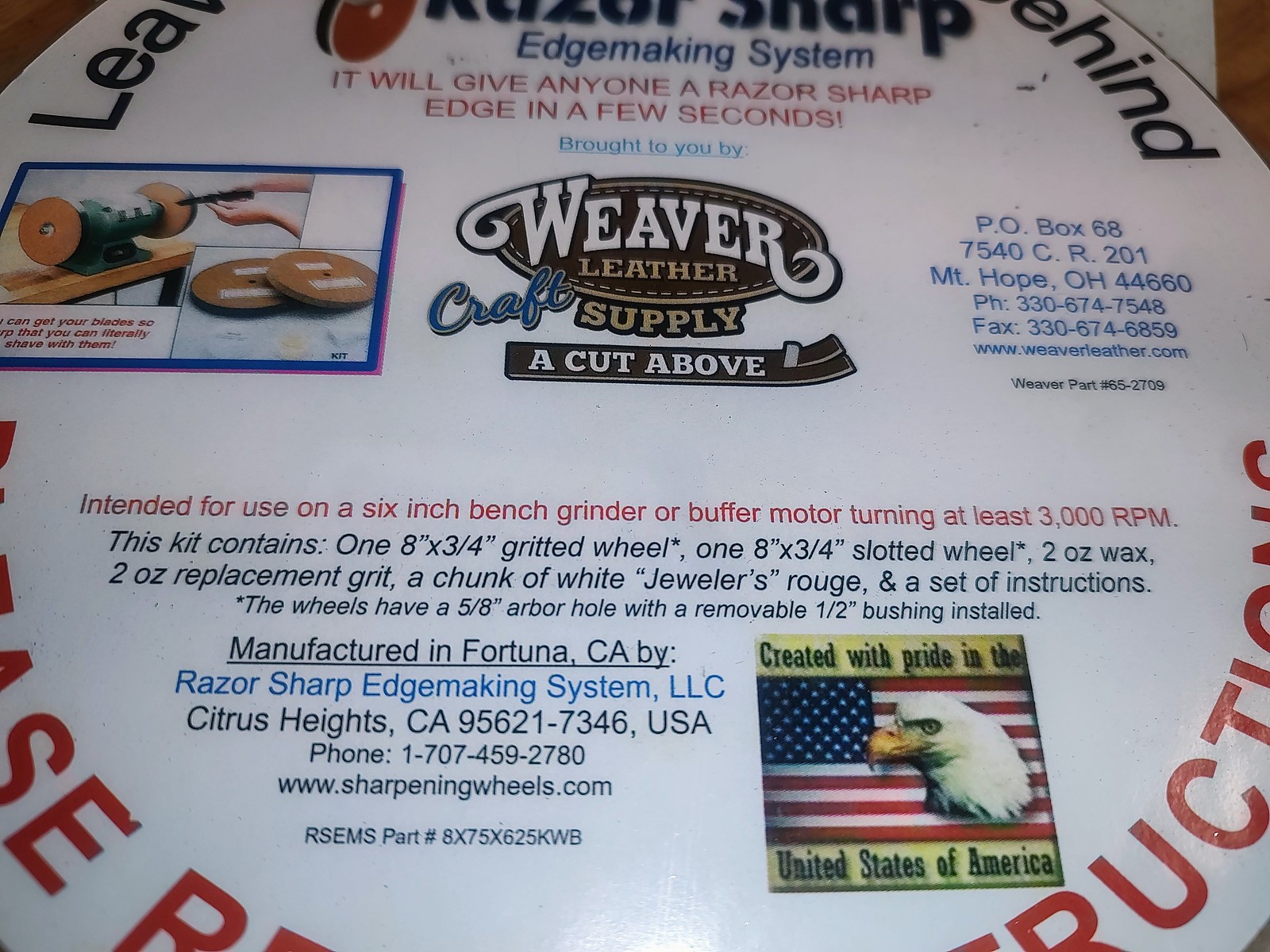The image features a detailed label from a product packaging for the "Weaver Leather Craft Supply Cut Above." The central part of the label previously displayed a white circle with the product name prominently written. Above this, it read "Razor Sharp Edge Making System."

To the right of the label, there was printed information including the address: "P.O. Box 687, 540 CR 201, Mt. Hope, OH 44660", followed by contact numbers: "330.674.7548" and "Fax: 330.674.6859." The website "www.weaverleather.com" is also listed for additional inquiries.

On the left side of the label, it mentioned illustrations of someone sharpening a tool. The label detailed the intended use of the product, stating it is designed for a 6-inch bench grinder or buffer operating at 3,000 RPM. The kit comprises one 8-inch by 3/4-inch graded wheel, one 8-inch by 3/4-inch slotted wheel, a two-ounce container of wax, a two-ounce container of replacement grit, a wide tool-edge router, and a comprehensive set of instructions. Both wheels feature a 5-inch arbor hole.

Additionally, the manufacturing information indicated that the product is manufactured in Fortuna, CA by Razor Sharp Edge Making System LLC, with a further reference to "Heintz, CA" and the website "www.sharpener.com."

This label provides detailed information about the product, its components, and contact details for customer inquiries.